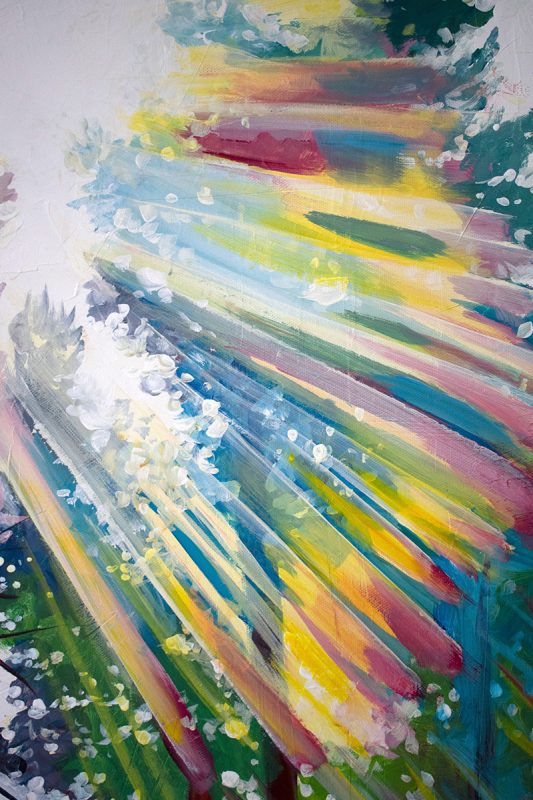This oil painting depicts an abstract representation of sunbeams piercing through a forest. The top left corner is dominated by a gray-white light, from which numerous streaks of paint—ranging in color from pink, yellow, and light blue to red—radiate across the canvas in a sweeping arc that extends to the bottom center and top right. These beams of color seem to distort the forest behind them, causing the leaves and trees to appear in shades of light blue, green, and other hues. The central tree is particularly noteworthy, with its light blue leaves suggesting the transformative effect of the sun's rays. While the bright blue and green background further enhances the vibrant atmosphere, delicate white specks scattered throughout the painting add a sense of ethereal detail, capturing the essence of a sunburst at early sunrise or nearing midday. The overall effect is a mesmerizing blend of natural beauty and abstract artistry.